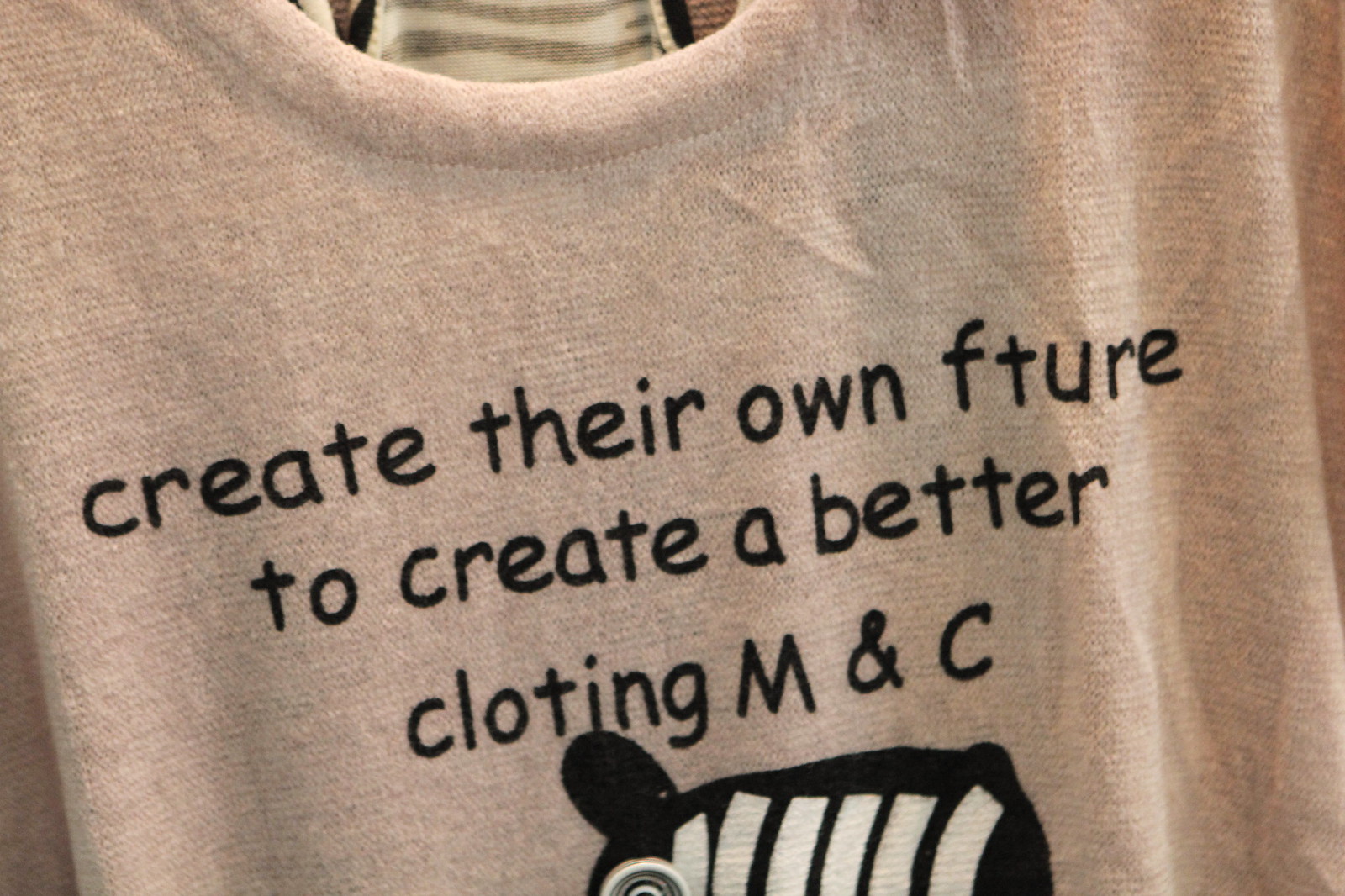This image showcases a light pink, slightly wrinkled t-shirt featuring a creative slogan and a partly visible black and white logo. The slogan, written in small black font, reads "create their own F T U R E to create a better CLOTHING MNC," with the letter "U" in "FUTURE" missing. Below the text is a black and white graphic, possibly depicting a zebra head pointing towards the right. The label inside the shirt is visible, positioned against an indistinct background. Additionally, the collar area and the interior of the shirt show parts of black and white stripes.